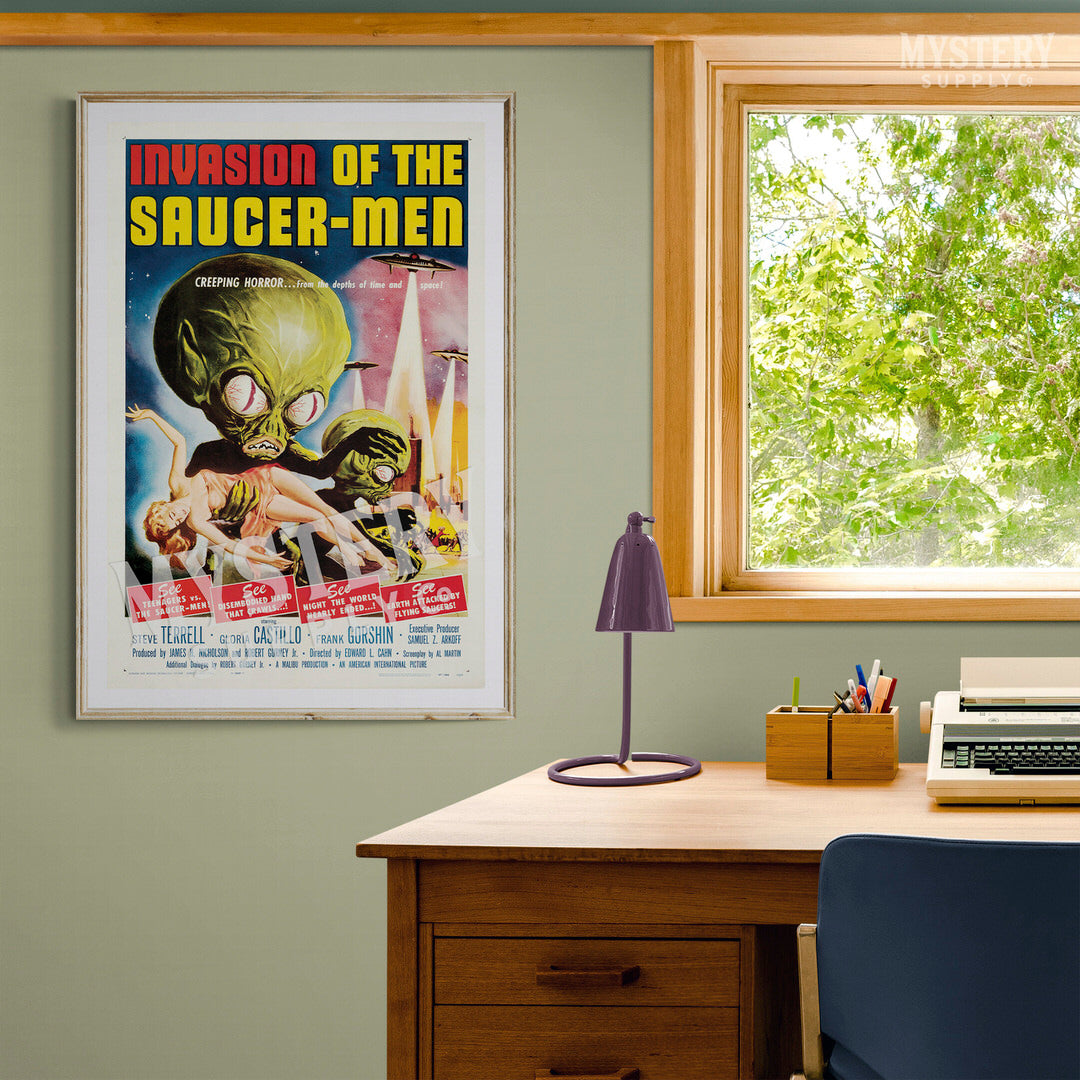A cozy little desk area is set against a light gray wall with subtle light wood trim. Dominating the wall is a large, eye-catching poster with retro sci-fi flair titled "Invasion of the Saucerman." The title "Invasion" is boldly rendered in red, while "of the Saucerman" stands out in yellow. The poster features a striking image of a green alien with large, white eyes that have vertical slits, and massive hands, with the word "Mystery" emblazoned across it. The bottom of the poster is accented with red hues. Below this vibrant artwork rests a neatly organized desk crafted from light brown wood. A comfortable blue chair is tucked under the desk, complemented by a vintage white typewriter. Also adorning the desk are a couple of small wooden boxes filled with pens and a petite purple lamp, adding a whimsical touch to the workspace.